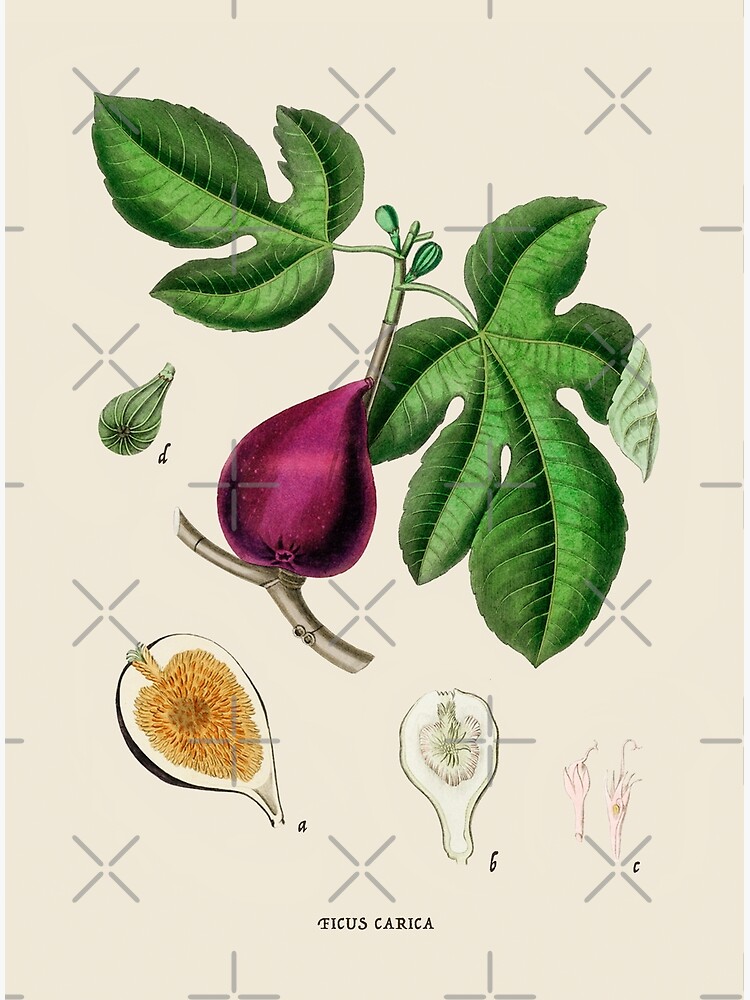This is a detailed and colorful botanical illustration labeled "Ficus carica," set against a pale tan background featuring a pattern of repetitive, slightly separated gray X's. The main focal point is a vivid, maroon fig with a magenta hue, depicted with great detail. The fig features a brown stem at the top, leading to two large green leaves—one with three stems, the other larger with five. Beyond the central fig, the illustration includes additional views: an immature green fig in the upper left corner, and multiple depictions of the fruit's interior below and to the left. These additional views include a vibrant color cross-section highlighting the magenta flesh and orange-hued interior, a black-and-white section, and a faint pink blossom representing the fig's flowering stage. Beneath the main fig, a brown branch extends, and the detail of one leaf's underside is shown. The entire composition, resembling a page from a botanical book, provides a comprehensive look at the fig's external and internal structure.